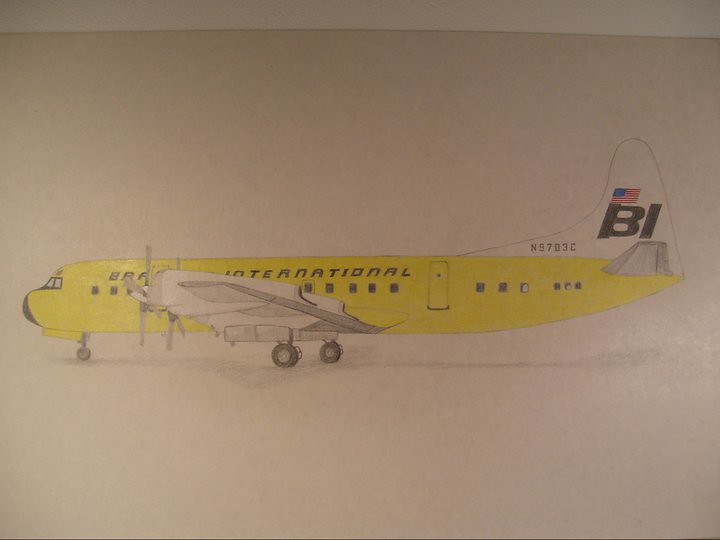This detailed pencil drawing features a propeller-driven aircraft depicted from a left side view on a plain white sheet of paper. The aircraft's fuselage is vividly colored in a school bus yellow, contrasting with the white left wing that houses two engines, each equipped with propellers. The rear vertical stabilizer (tail wing) is also white, adorned with a detailed representation of the USA flag, featuring blue, red, and white stars and stripes. Below the flag, the initials "BI" are boldly inscribed in black. The tail wing also displays the registration number "N57B3C" in black lettering. Additional details include the aircraft's black nose and visible landing gear with three wheels extended.